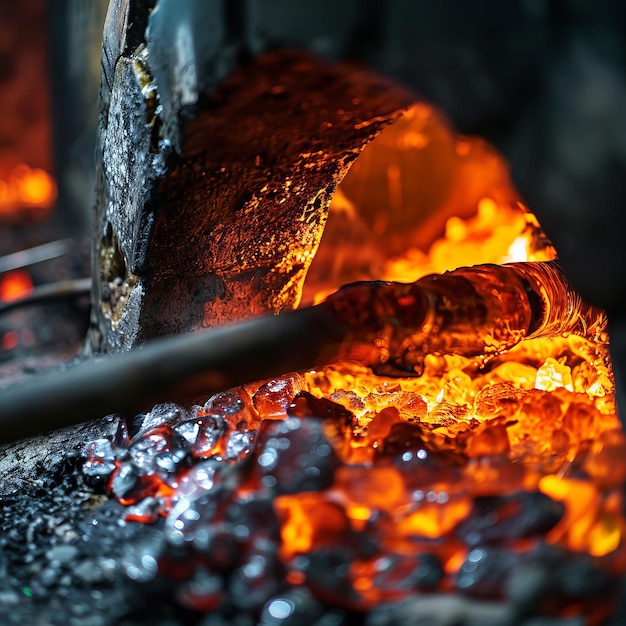This photograph captures a close-up view of a glowing furnace, likely used in blacksmithing or glassworking. The image prominently features a dark stone arch, marking the entryway into the furnace. Below the arch, an intense bed of coals transitions from black at the edges to vibrant red, yellow, and orange hues toward the center, indicating the extreme heat. A steel rod, possibly a fire poker or tool, extends from the left side of the photograph into the heart of the furnace, with sparks and embers visibly dancing around it. The bottom of the scene showcases scattered rocky debris, which further enhances the rugged and fiery environment of this industrial kiln.